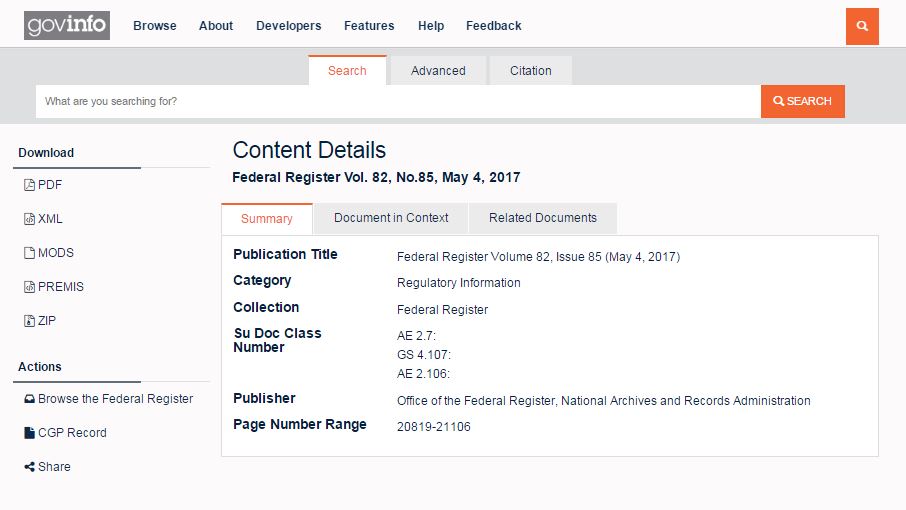This is a screenshot from GovInfo. At the top left corner within a gray box is the GovInfo logo. To its immediate right, across the top header, there is a menu bar with the following options: Browse, About, Developers, Features, Help, and Feedback. On the far right of this same row, there is an orange search button. 

The header consists of two sections: the upper section contains the menu and search button, while the bottom section has a light gray background and features three tabs above a search bar. These tabs are labeled Search, Advance, and Citation. To the end of the search bar on the right side, there is another orange search button.

Below the header, the main content of the page includes a sidebar with two sections labeled Download and Actions. On the right side, the primary content area is titled "Content Details" with a smaller subtitle specifying "Federal Register Volume 82, Number 85, May 4, 2017." Beneath this title is a white chart with three tabs: Summary, Document and Context, and Related Documents. The visible content shows the Summary tab, which contains approximately five to six rows of information including the publication title "Federal Register Volume 82, Issue 85 for May 4, 2017," as well as additional details such as category, collection, SUDOC class number, publisher, and page number range.